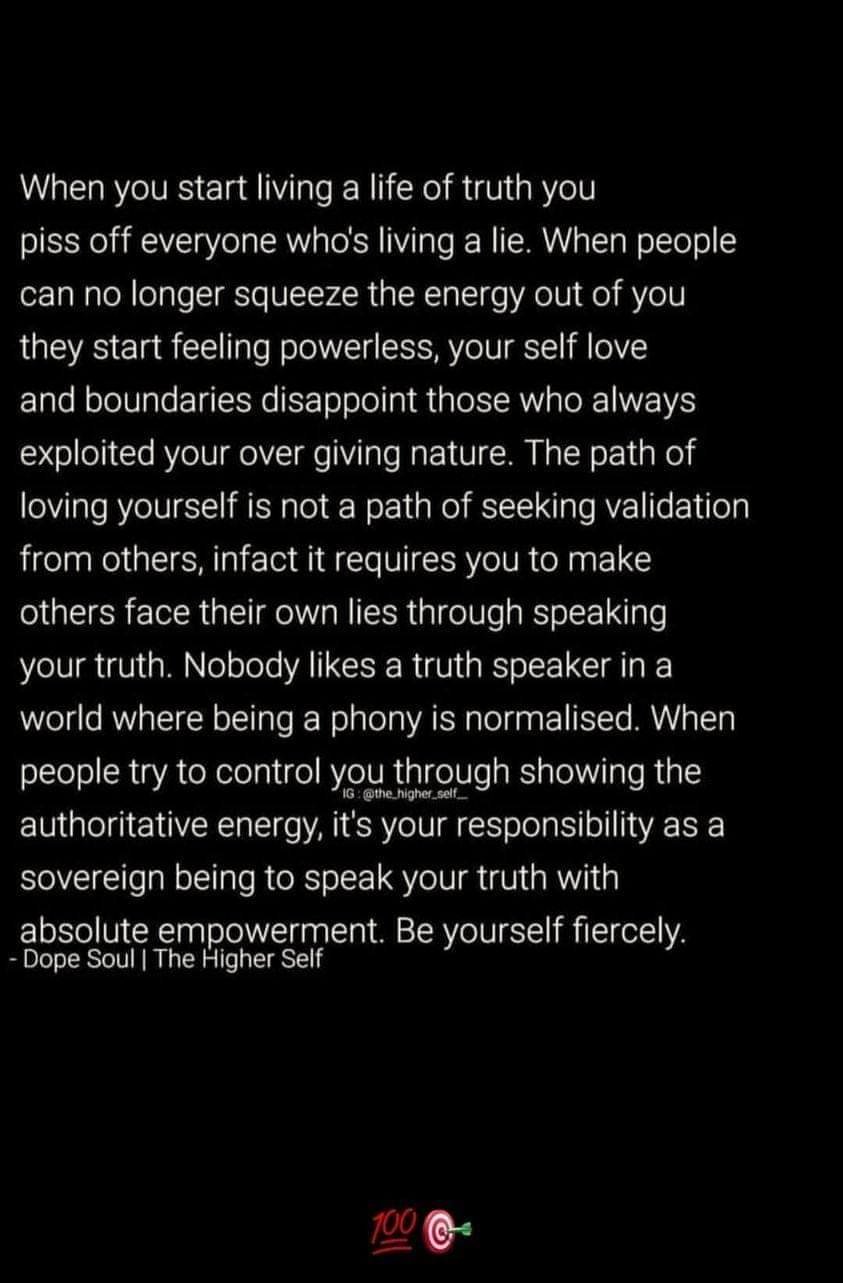The image features a striking design with white text against a solid black background, arranged in left-justified lines. At the bottom of the image, there is a colorful design element: a red number "100" that is double-underlined, alongside a red and white circular target with a green arrow piercing the bullseye. The text is an empowering quote attributed to "Dope Soul, The Higher Self." The quote reads: 

"When you start living a life of truth, you piss off everyone who's living a lie. When people can no longer squeeze the energy out of you, they start feeling powerless. Your self-love and boundaries disappoint those who always exploited your overgiving nature. The path of loving yourself is not a path of seeking validation from others. In fact, it requires you to make others face their own lies through speaking your truth. Nobody likes a truth speaker in a world where being a phony is normalized. When people try to control you through showing the authoritative energy, it is your responsibility as a sovereign being to speak your truth with absolute empowerment. Be yourself fiercely."

In the middle of the image, on the fourth line, the Instagram handle "@the_higher_self_" is displayed, indicating the source of the quote.